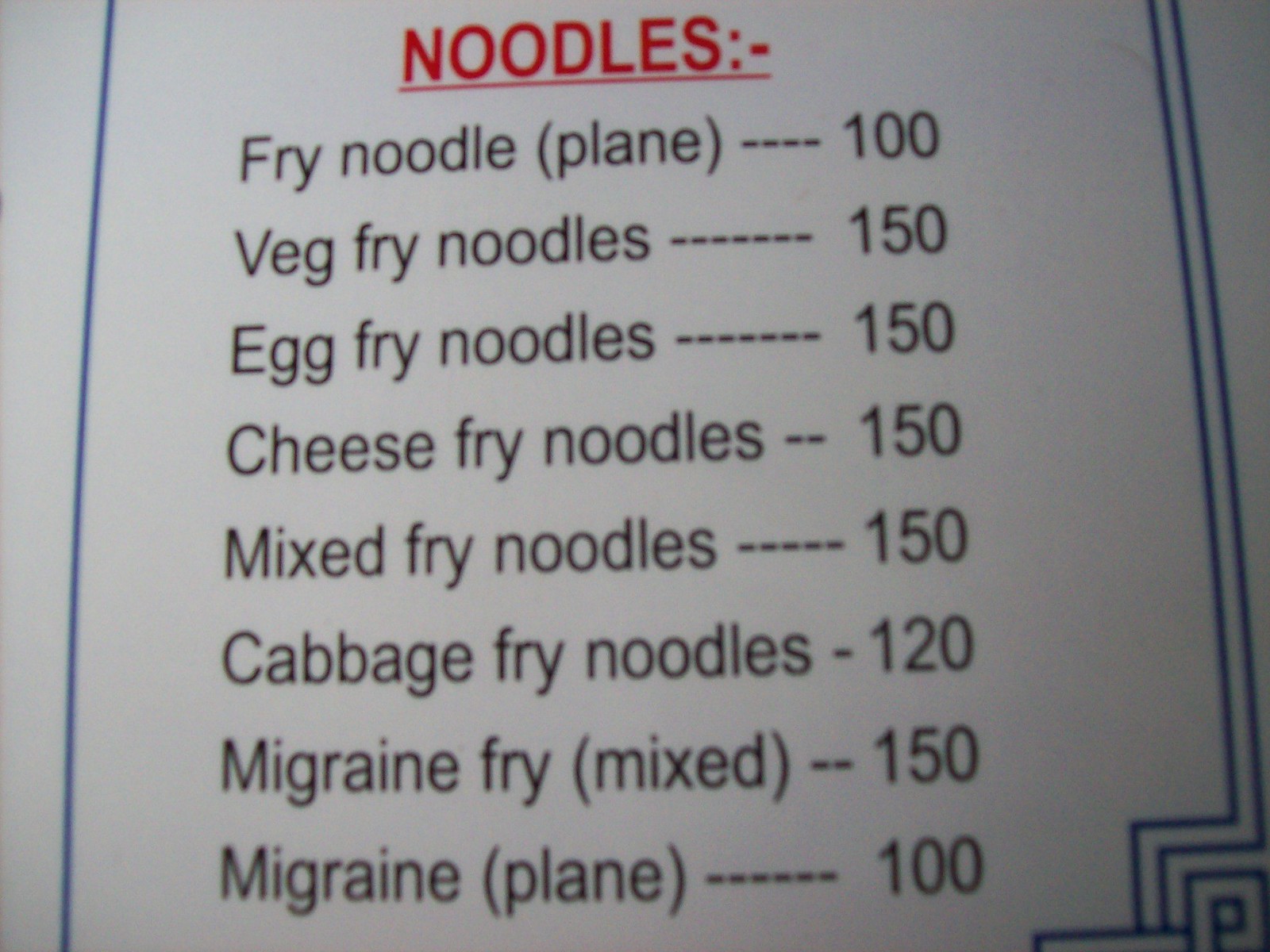The image showcases a detailed section of a restaurant menu against a white background, bordered by blue lines. A thin blue line runs vertically down the left side, while two similar lines run down the right, converging with additional lines to form a blue square with a smaller square inside, suggesting a corner section of the menu with a unique overlapping design. At the top center of this menu section, the word "NOODLES" is prominently displayed in bold, red, all-capital letters, underlined with a thin red line. Below this header, various noodle dishes are listed in black text alongside their prices, with notable items like "Fried Noodle [Plain (incorrectly as P-L-A-N-E)]" for 100, "Veg Fried Noodles" for 150, "Egg Fried Noodles" for 150, "Cheese Fried Noodles" for 150, "Mixed Fried Noodles" for 150, "Cabbage Fried Noodles" for 120, "Migraine Fry [Mixed]" for 150, and "Migraine [Plain (incorrectly as P-L-A-N-E)]" for 100. The image itself appears slightly fuzzy and out of focus.